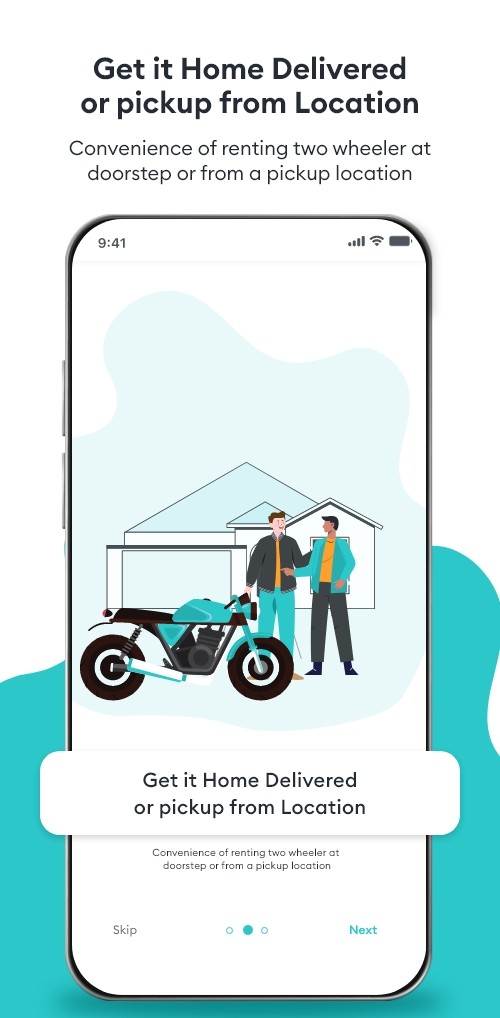A detailed illustration of a smartphone display features a delivery app interface for renting two-wheelers. Above the smartphone, bold text reads, "Get it home delivered or pick up from location," emphasizing the dual options available for renting. The main image within the screen showcases a cartoonish scene set in a suburban neighborhood: two individuals stand in front of a house, with one of them holding a motorcycle with an aqua or teal hue parked beside them. This depiction clearly conveys the convenience of either doorstep delivery or pick-up services for renting motorcycles or mopeds.

The text at the bottom mirrors the top message, reiterating the two rental options. The user interface includes navigational cues for swiping left or right, indicating additional informational pages on either side. A "Skip" button allows users to bypass the introductory content, while a "Next" button guides them through the slides. The app's background palette consists of predominantly white and light gray shades, providing a clean and modern look.